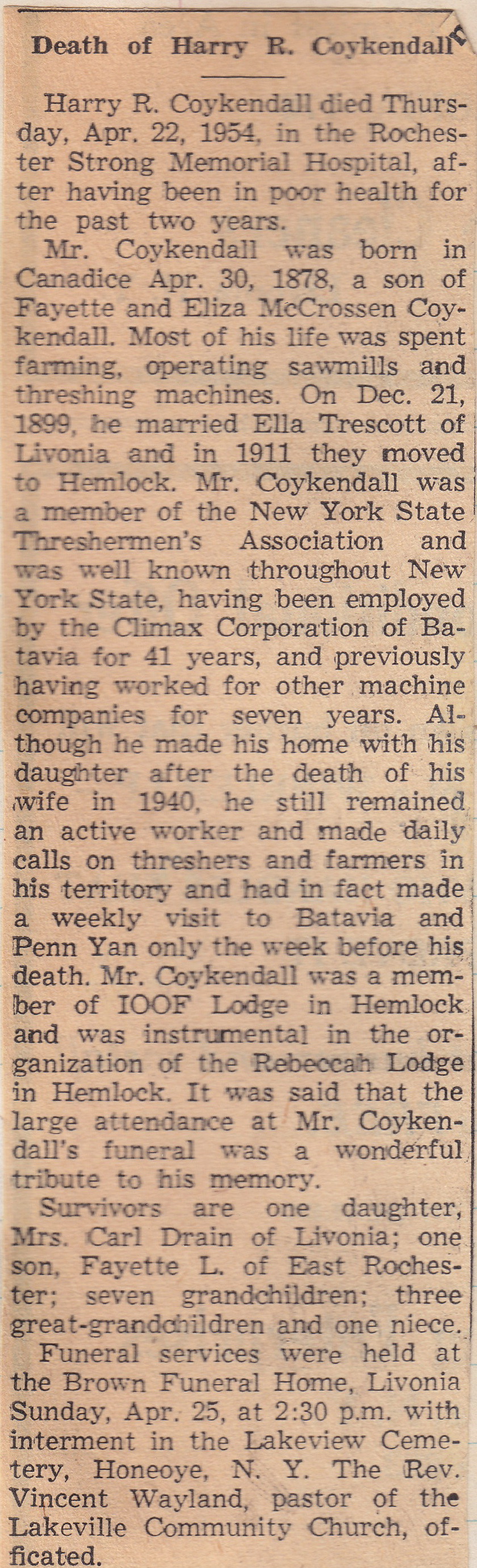This image is a slightly faded and yellowed vertical newspaper clipping of an obituary titled "Death of Harry R. Koykendall." The obituary announces that Harry R. Koykendall died on Thursday, April 22, 1954, in the Rochester Strong Memorial Hospital after having been in poor health for the past two years. Born in Canada on April 30, 1878, to Fayette and Eliza McCrossin Koykendall, most of Harry’s life was spent farming, operating sawmills, and threshing machines. He married Ella Trescott of Livonia on December 21, 1899, and in 1911 they moved to Hemlock. The obituary notes that Harry was a member of the New York State Threshersmen Association and was well-known throughout New York State for his work with the Climax Corporation of Batavia, where he was employed for 41 years.

After his wife’s death in 1940, Harry lived with his daughter but remained an active worker, making daily calls on threshers and farmers in his territory and even visiting Batavia and Pen Yen the week before his death. He was a member of the IOOF Lodge in Hemlock and helped organize the Rebecca Lodge there. The obituary adds that the large attendance at his funeral was a wonderful tribute to his memory. Harry is survived by one daughter, Mrs. Carl Drain of Livonia; one son, Fayette L. of East Rochester; seven grandchildren; three great-grandchildren; and one niece. His funeral services were held at the Brown Funeral Home in Livonia on Sunday, April 25, at 2:30 p.m., with interment in the Lakeview Cemetery, Oneye, NY, and officiation by Rev. Vincent Whalen, pastor of the Lakeville Community Church.